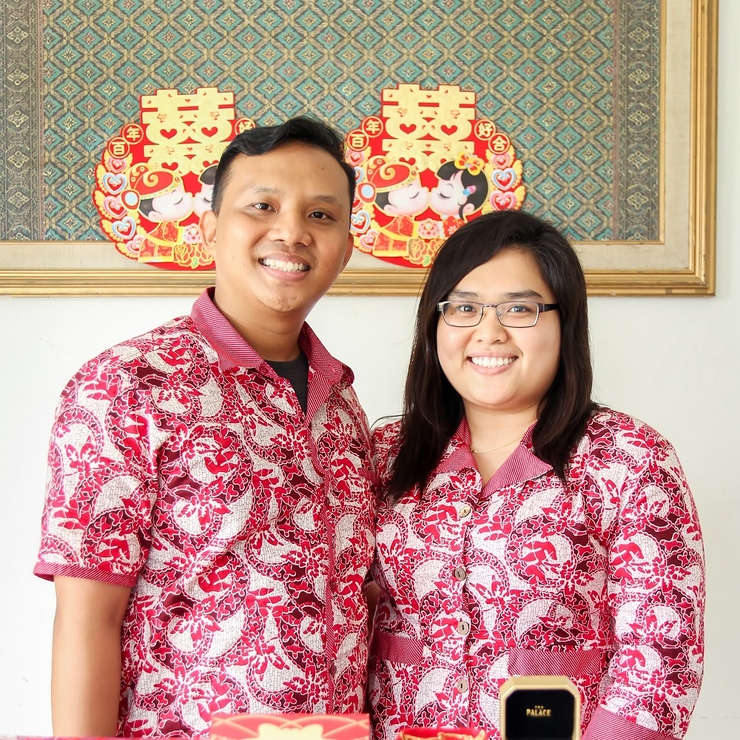A photograph features a smiling man and woman of Asian descent, standing side by side and facing the viewer as if posing. Both are dressed in matching button-down shirts adorned with intricate leaf and dragon-like designs in various shades of red, gray, and pink, with finely lined collars accentuating the ensemble. The woman, distinguishable by her shoulder-length hair, glasses, and round face, stands to the right of the taller man. They are positioned against a plain off-white wall, adorned with a framed piece of art. This artwork, appearing to be textile or fabric, showcases two cartoon-like figures kissing. Accompanying the central image are two decorative banners featuring Asian script, hearts, and additional images of the kissing figures, one with a flower in their hair and the other with a red hat, evoking a sense of a loving or celebratory theme, possibly reminiscent of Valentine's Day.